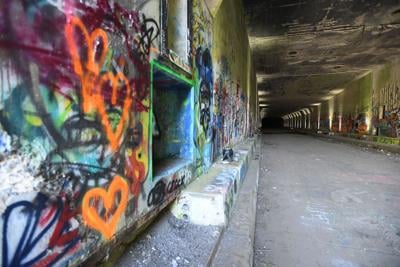This photograph captures the entrance of a graffiti-laden tunnel in a big city, possibly underneath a bridge for car overpass. The tunnel's gray concrete floor, walls, and ceiling are adorned with a vibrant array of graffiti that extends all the way down its length. Notably, the left wall, being closer to the camera, showcases an intricate tapestry of street art, including prominent orange hearts, a black spray-painted face, and a human skull. Accompanying these are splashes of black, red, and blue, including blue paint within what appears to be a spillway for water. The right wall and ceiling also host graffiti, although the details become indistinct as they recede into the tunnel's depth. Illuminated by overhead lights, the tunnel appears to narrow and darken as it stretches deeper, creating a compelling sense of depth and mystery. Despite the saturation of artwork, no identifying information, such as the tunnel's location or construction date, is visible in the image.